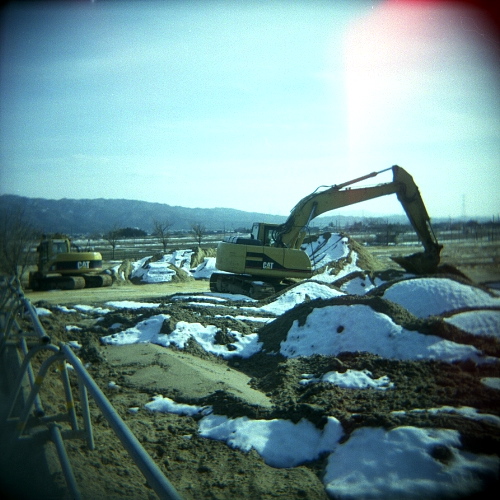The image is a rectangular, vintage-style photograph depicting a construction site with a noticeable reddish glare in the top right corner, indicating a camera imperfection. The colors appear dull and the overall hue has a greenish-blue tint, reminiscent of older photographs. The outdoor scene occurs during a colder season, evidenced by thin patches of snow dusting the piles of dirt scattered around. In the foreground, there are several large pieces of heavy machinery, including a yellow and black backhoe with a scooping bucket and another similar piece of construction equipment, both branded with the CAT symbol. To the left, there's also a chain-link fence, broken up with visible metal poles, serving as a boundary to the site. The backdrop of the image features a landscape with a low mountain range that gradually rises from right to left. The sky is a mix of brightish blue and gray, contrasting with the earthy hues of the construction site below.